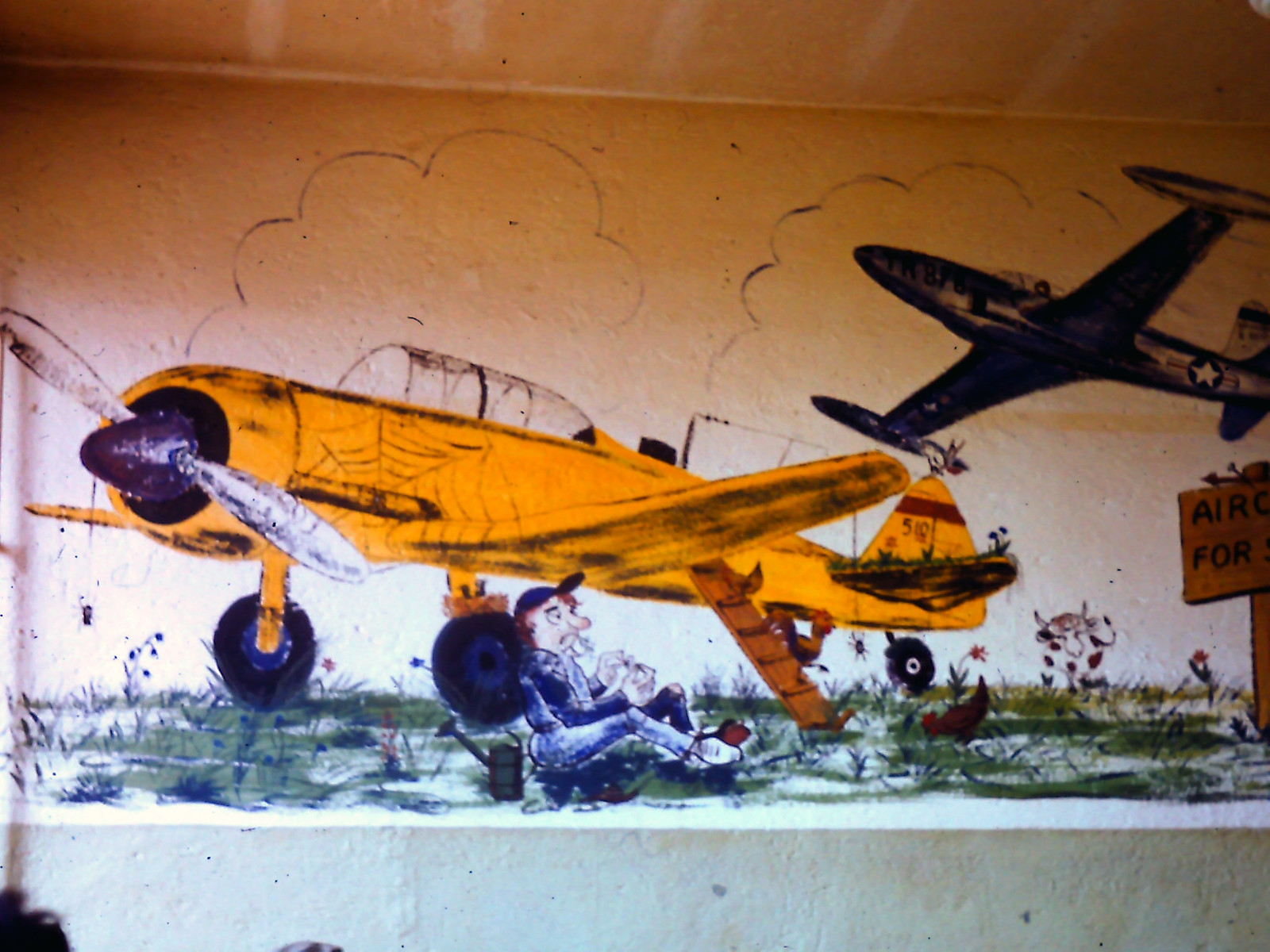The image depicts a cartoon-like drawing of two old-fashioned helicopters, surrounded by a mix of whimsical and realistic elements. Central to the image is a characteristically drawn man wearing a hat, casually sitting in a field with a chicken nearby. The man leans against the wheel of a yellow helicopter, which is grounded amidst grassy terrain. A few other animals are also depicted roaming around on the ground. 

In the sky, a second helicopter, blue with a white star near its tail, is seen flying against a backdrop of two abstract clouds. The setting includes a hand-drawn wooden sign that reads "Air for," combining both literal and playful textual elements. The overall background of the image is white, with the color palette featuring an abundance of yellows, whites, blacks, blues, reds, and touches of gray. This vibrant illustration, marked by its casual and charming style, captures a scene rich with detail and a sense of playful leisure.